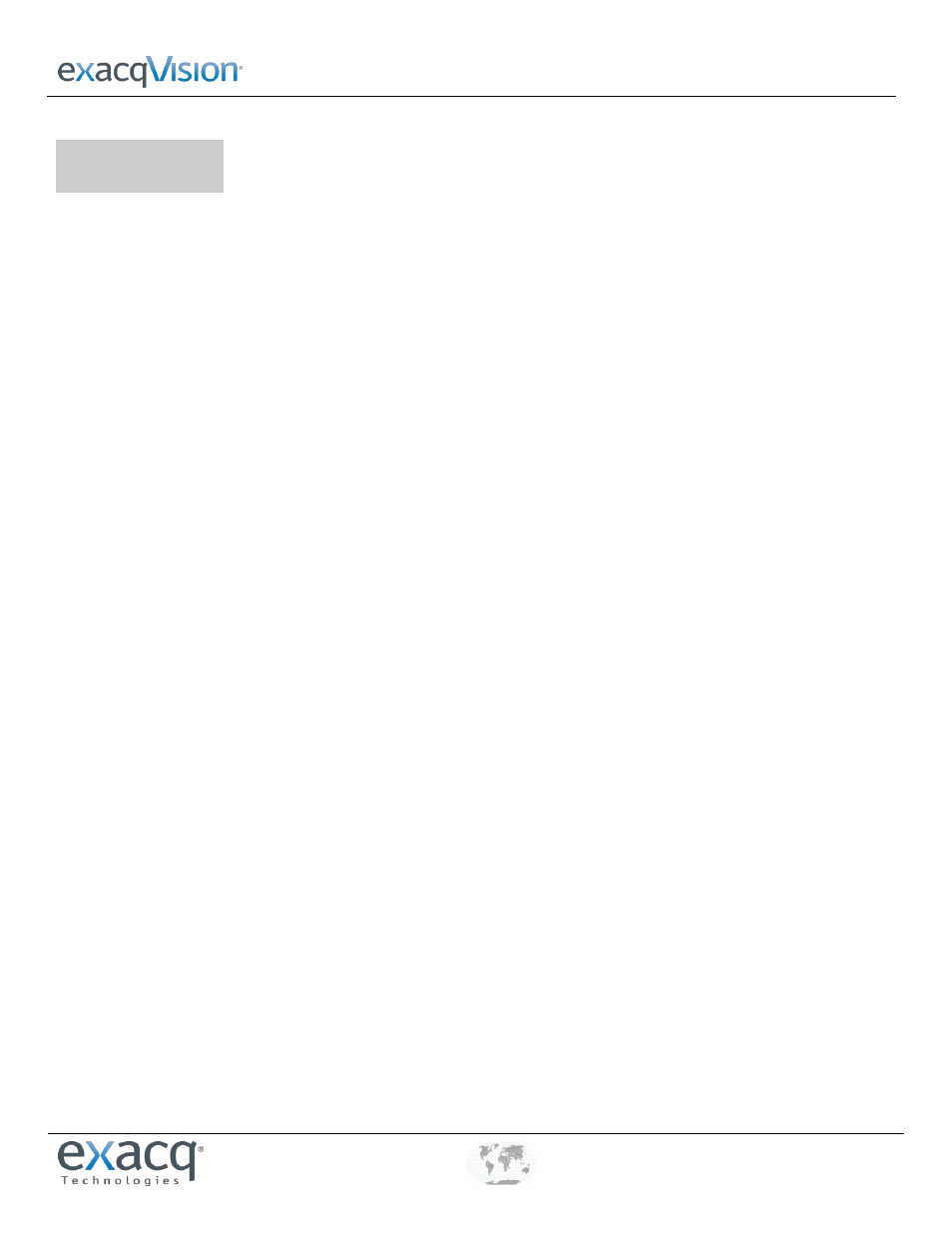The image features the text "Exacq Vision," with "Exacq" spelled as "E-X-A-C-Q," where the "X" is a light blue color and the remaining letters are a dark blue. The word "Vision" follows in all dark blue letters, except for the initial "V" which is capitalized and in dark blue. There is an underline beneath "Exacq Vision." 

Towards the bottom of the image, the text "Exacq Technologies" appears, again with the "X" in "Exacq" colored light blue and the other letters in dark blue. A horizontal black line is positioned above this text. The rest of the image is blank, with a gray box present that is not labeled. 

The minimalist color scheme of dark and light blue combined with the structured layout creates a professional and sleek appearance.